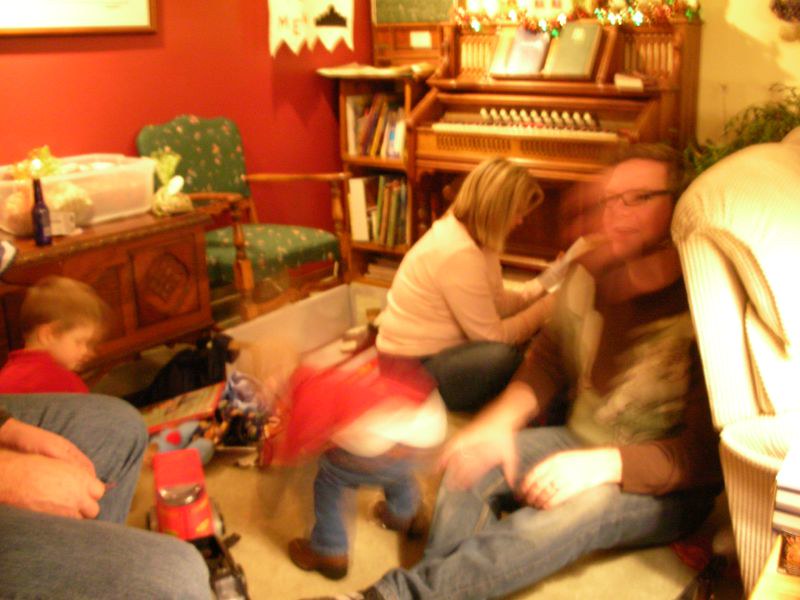In a cozy, lived-in home, the scene captures a bustling family moment. At the center, a white adult male with light brown hair and square-framed glasses sits on the floor in blue jeans and a brown sweater adorned with a Christmas tree design. He is smiling or mid-sentence, his facial expression full of warmth. Beside him, another white adult, a woman with dirty blonde, mid-length hair styled in a bob, is also dressed in blue jeans paired with a white long-sleeved shirt. She seems engaged in reading something unidentifiable.

In front of them, two young children are absorbed in play. One child, wearing a red shirt, is focused on toys scattered around. The second child, in a red-and-white shirt and blue jeans, is caught in motion, perhaps bending toward the floor to reach another plaything. Both children, like the adults, are slightly blurred, hinting at the lively chaos of the moment.

An additional adult, only partially visible by their hands and feet, sits across from the man, suggestively similar in attire with blue jeans. Scattered around are various toys, including a notable red truck. The background adds more color to the narrative: Christmas decorations or similarly festive decor, a bottle of beer perched on a wooden chest, and a wooden chair with a green, flower-patterned seat. A vintage wooden piano with books lined beside it adds a nostalgic touch. Partially visible next to the man is a beige or cream couch, further emphasizing the warm, inviting nature of the space.